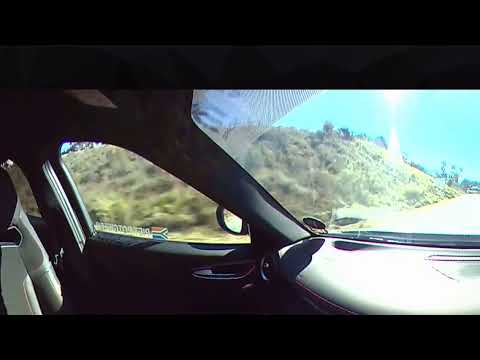The image captures the interior of a car with a grayish color scheme, including dark and light gray elements. The dashboard features a slight brown trim and racer seats in gray and black are visible. You can see the handle doors, the driver's side mirror, and a partial view of the seat. The window has a decal featuring the South African flag in red, white, blue, and black, along with unreadable white text. The windshield has another dark-colored sticker. Through the windshield, the sun is shining brightly, casting a glare that makes some details harder to see. Outside, the road is flanked by a hill covered in green vegetation and small bushes. The sky is vividly blue, indicating clear weather. The setting confirms that the car is in motion, driving along a roadway bordered by natural greenery.